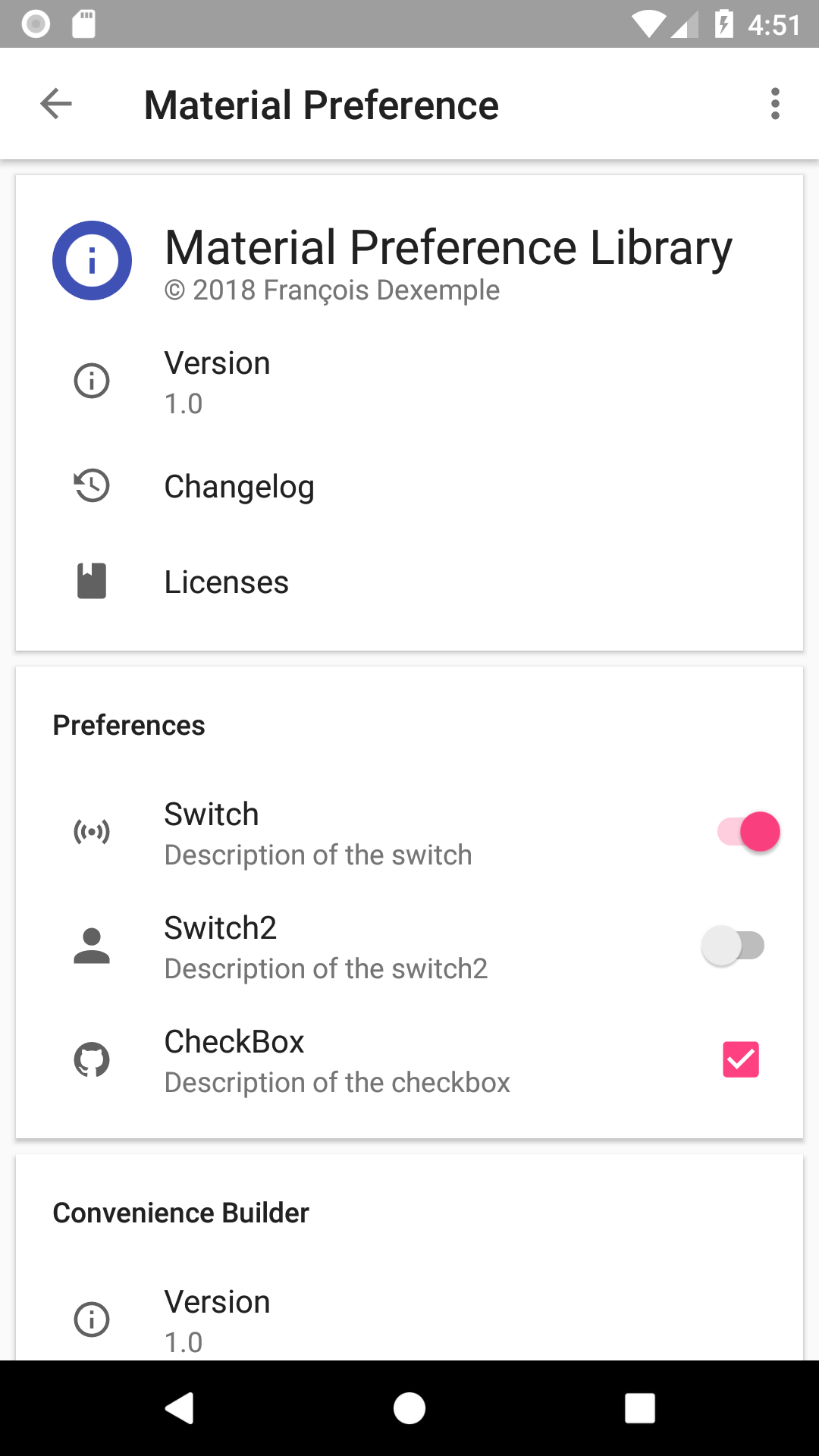The screenshot image displays a detailed user interface of a mobile application. In the top right corner against a gray background, it indicates the time as 4:51, a full battery icon, and a Wi-Fi signal. Below this, on a white background in black text, the label "Material Preference" is shown with a left-pointing arrow. 

Further down, enclosed within its own white box, the interface lists the following entries: "Material Preference Library," "2018 Copyright Francois D'Exemple," "Version 1.0," "Change Log," and "Licenses."

Continuing below, another rectangular section labeled "Preferences" is visible. Under "Preferences," there is a labeled switch with a description beside it. The toggle switch is red and turned on. This is followed by a second switch, "Switch to," also accompanied by a description.

Below the switches, there is a checkbox with its corresponding description. The checkbox is marked with a white check in a red box to the right. 

Finally, at the bottom of the image, the text reads "Convenience Builder Version 1.0."